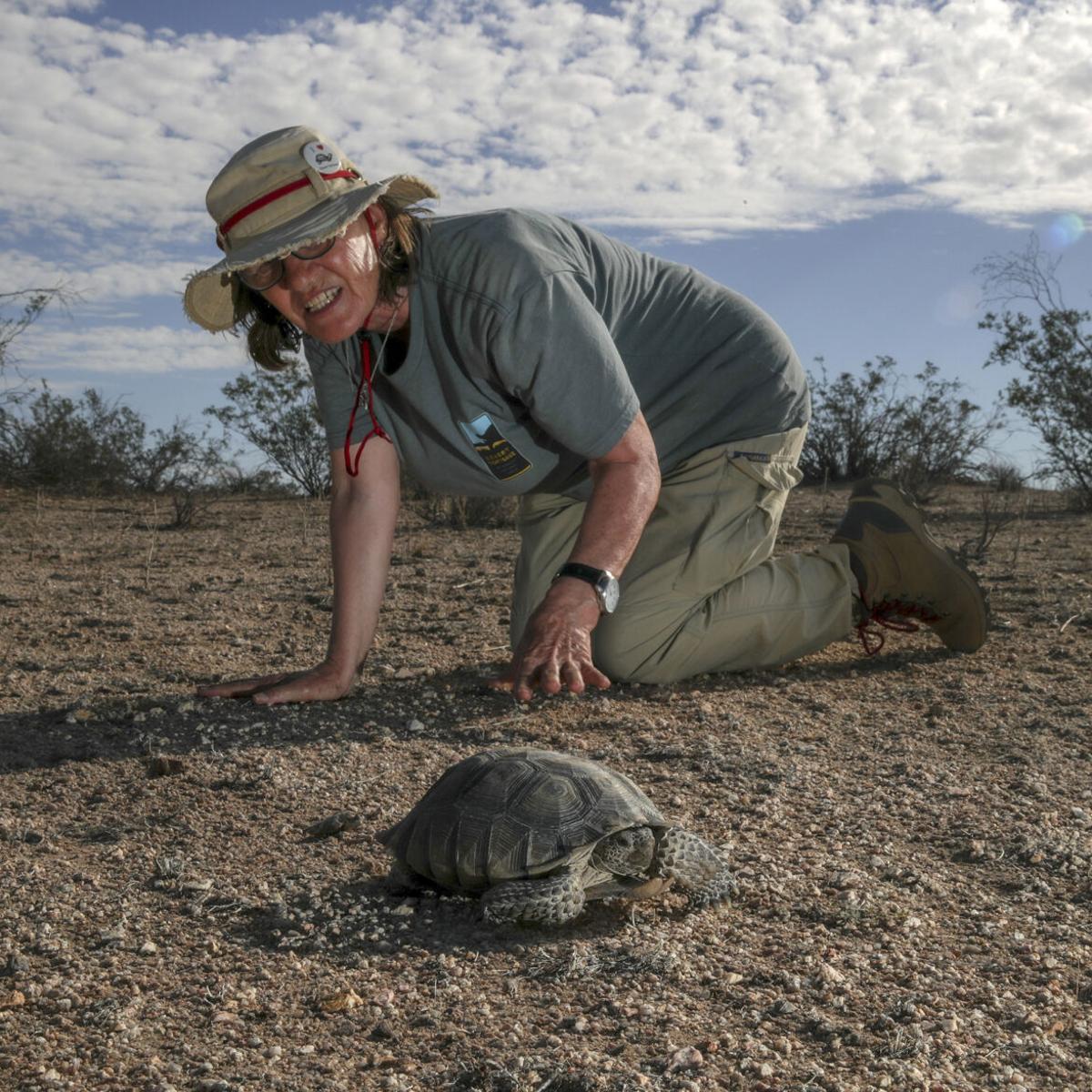In this vivid outdoor photograph, a person dressed in khaki pants, a gray short-sleeve shirt, and brown hiking boots is kneeling on a dirt and gravel surface, their right hand supporting them while their left hand, adorned with a watch, reaches out towards a turtle. The person's gender is ambiguous, but they have brown hair and are wearing glasses beneath a tan bucket-style hat with a red ribbon and a noticeable pin attached to it, partially obscuring their eyes. They are staring intently at the turtle, with their mouth open and teeth clenched. The turtle, mostly retracted into its brownish-green shell, is positioned in the lower central part of the image with its head slightly visible. The background features a blend of sparse bushes and a beautiful, partly cloudy sky with feathery white clouds and patches of blue.